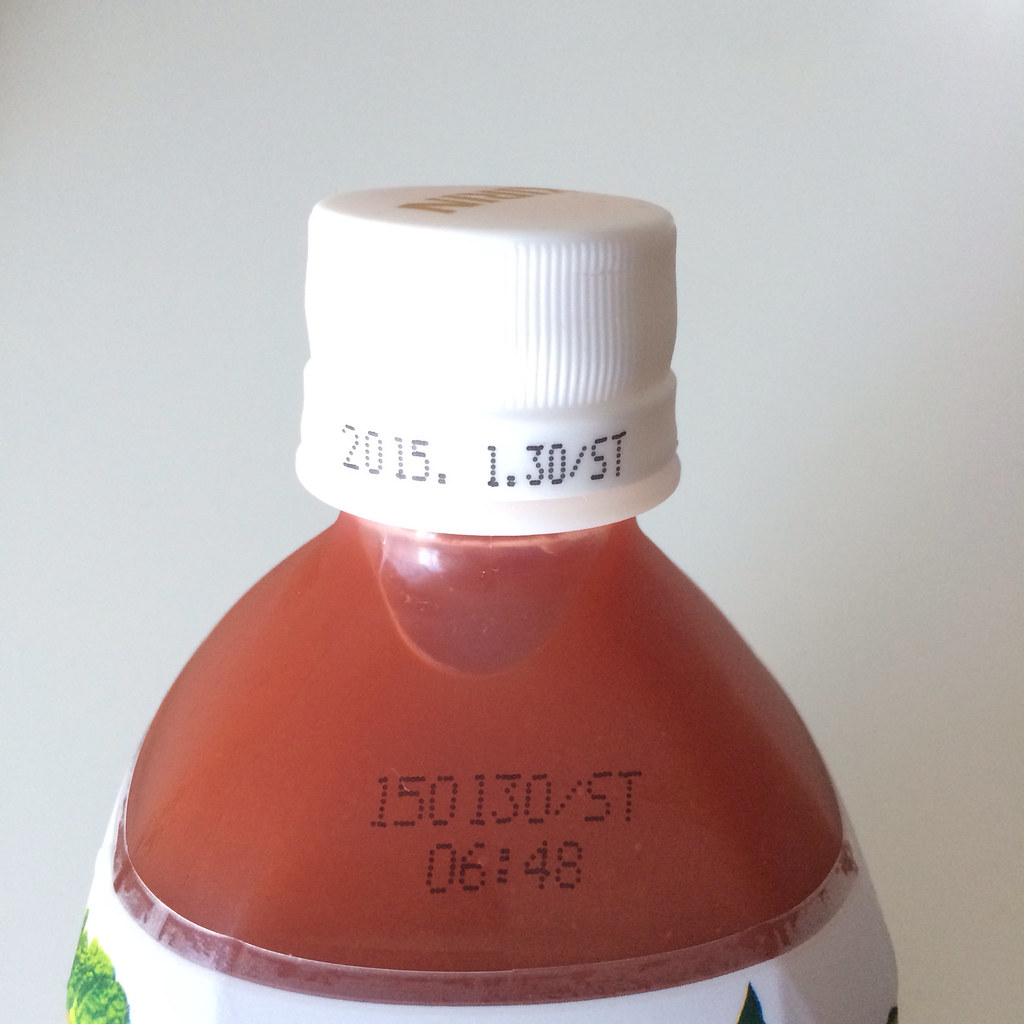This very close-up photograph captures the upper third of a plastic bottle containing a reddish liquid, likely a vegetable or fruit juice. The bottle is full and unopened, with an intact tamper-proof white screw cap. The top of the cap features gold-colored letters, although the exact text is obscured by the angle of the shot. Printed along the rim of the cap is a date code: "2015-130/ST." Additionally, other codes such as "150-130-ST" and "06-48" are visible around the neck of the bottle, suggesting manufacturing details. The bottle has a partial white plastic label wrapping around it, displaying green leaves, hinting at the natural contents of the juice. The overall background of the image is plain and gray, emphasizing the detailed textures and labels of the bottle itself.